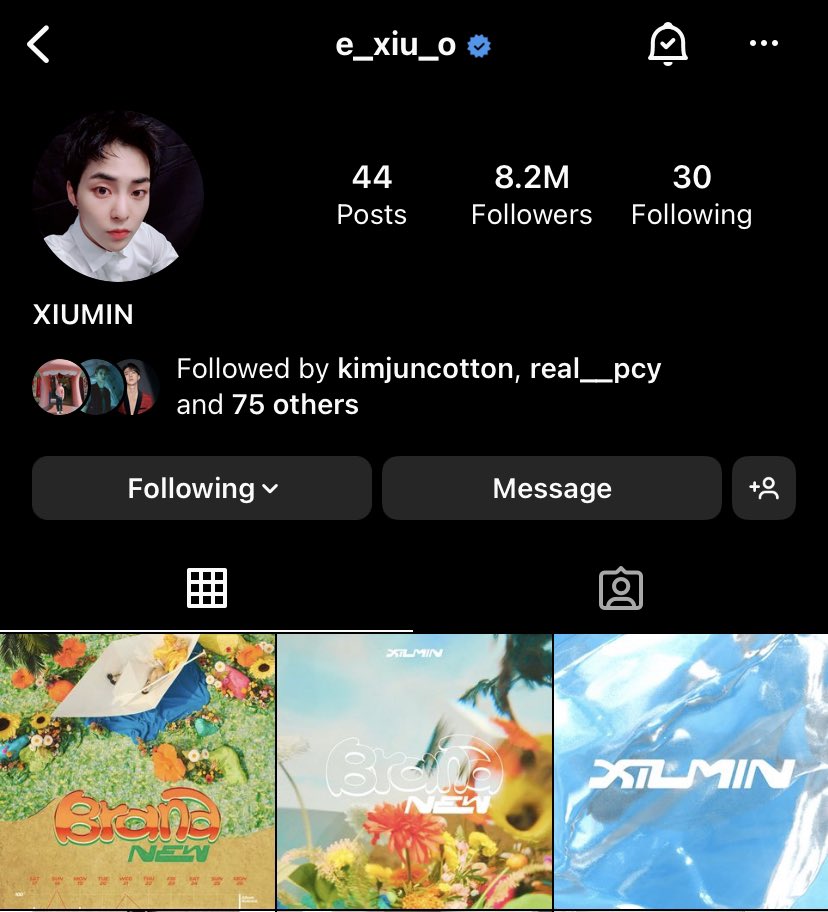Screenshot of Twitter profile of a popular androgynous Korean musical artist, known by the username XIUMIN, displayed in all caps. The profile picture shows a youthful person, whose gender is ambiguous, adding to their unique and intriguing persona. The artist boasts an impressive following with 8.2 million followers while following only 30 accounts and having posted 24 times. At the bottom of the screenshot are multiple album covers, hinting at their musical career. Among the visible album titles is "Brand New," written in a stylish font that is somewhat difficult to read. Notably, XIUMIN is followed by notable accounts such as KimJunCotton and RealPCY, alongside 75 others. The artist’s popularity is evident, although they may be unfamiliar to those outside this musical scene.